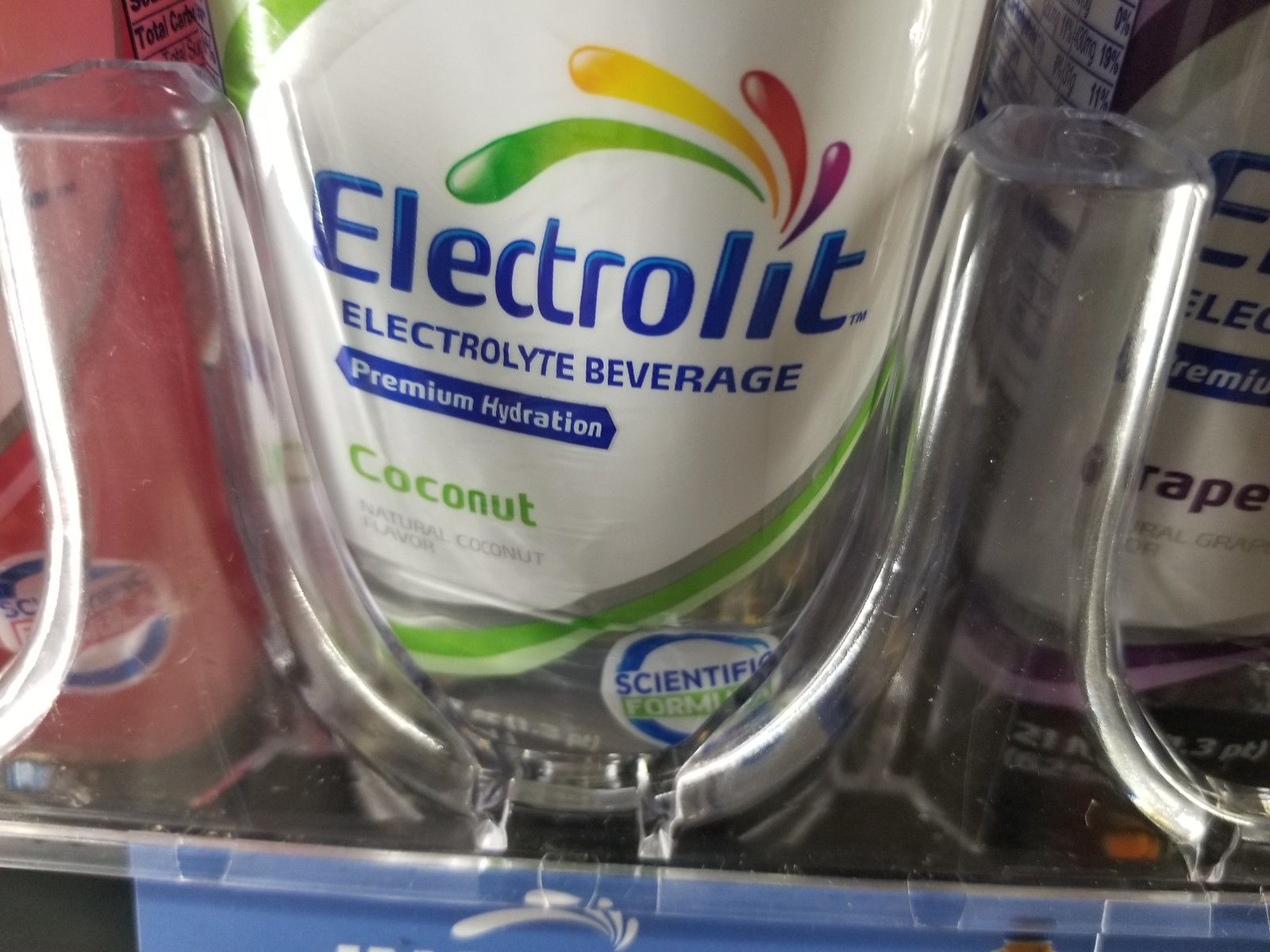The image displays a close-up view of a product inside a glass case typically found in convenience stores. The featured product is "Electro-Lit," an electrolyte beverage known for its premium hydration qualities. The focus is on a coconut-flavored variant, distinguished by a white label with green trim and the "Electro-Lit" logo featuring four halogenated droplets in green, yellow, red, and purple. The bottle itself is clear, allowing the contents to be visible. At the bottom of the bottle is a small sticker in blue, white, and green, indicating "scientific formula."

Adjacent to the coconut-flavored Electro-Lit, on both sides, are other flavors of the same product. On one side, the grape-flavored beverage is identifiable by its white label with purple borders. On the other side, you can partially see a bottle with pinkish contents, presumably another flavor variant, also marked by the "scientific formula" sticker at the bottom.

The bottles are secured on the shelf by clear plastic holders, which keep them in place. At the very bottom of the image, there is a glimpse of another label featuring part of the Electro-Lit logo in white, likely indicating the product's price.